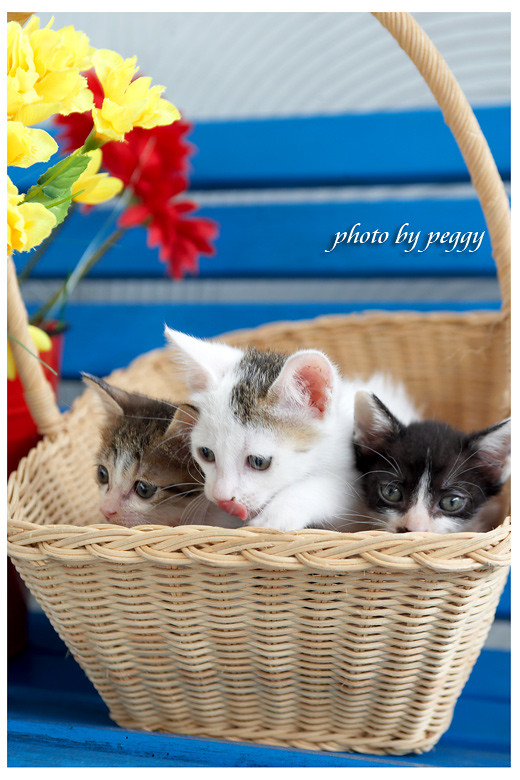This endearing image, taken by Peggy, features three adorable kittens nestled inside a woven wicker basket with a long handle. The basket is set atop what appears to be a blue desk or bench, complemented by additional blue lines in the background and some white areas at the top. To the left in the image, vibrant yellow and red flowers are visible, adding a splash of color to the scene. 

The kittens, all with striking green eyes, present a charming trio: the kitten on the left is a brownish-gray with little black stripes, the one in the middle is predominantly white with a distinctive black stripe on its head, and the one on the right has a black head with a contrasting white nose. They seem to be focusing their gaze towards the left side of the image, except for the black and white kitten on the right, who looks straight ahead. This heartwarming photograph beautifully captures the innocent curiosity of the kittens against a simple yet appealing backdrop.